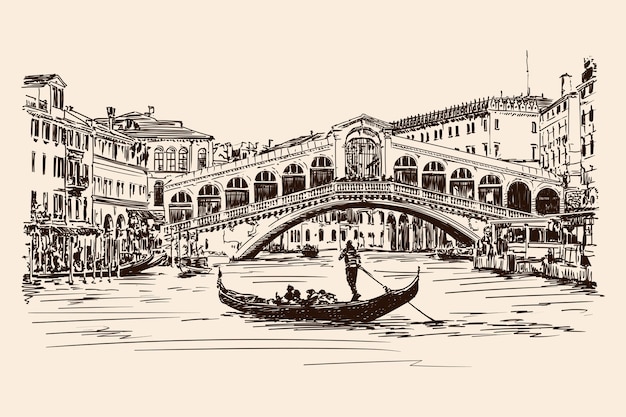This detailed black and white pen and ink illustration depicts a picturesque scene of Venice, Italy. The foreground showcases a traditional gondola navigated by a gondolier using a long paddle, with passengers seated inside, capturing the iconic Venetian charm. The waterway is lined with tall, ornate buildings that border a canal, reflecting the city's architectural splendor. A prominent feature of the scene is a covered, arched bridge adorned with stone decorations and trim, spanning the canal and connecting both sides. The bridge hosts tiny figures of people, adding a sense of scale and liveliness to the illustration. Additional boats are visible along the sides, suggesting a bustling yet serene waterway. The image is a meticulously detailed pencil drawing, with no textual elements, emphasizing the timeless and tranquil beauty of Venice.